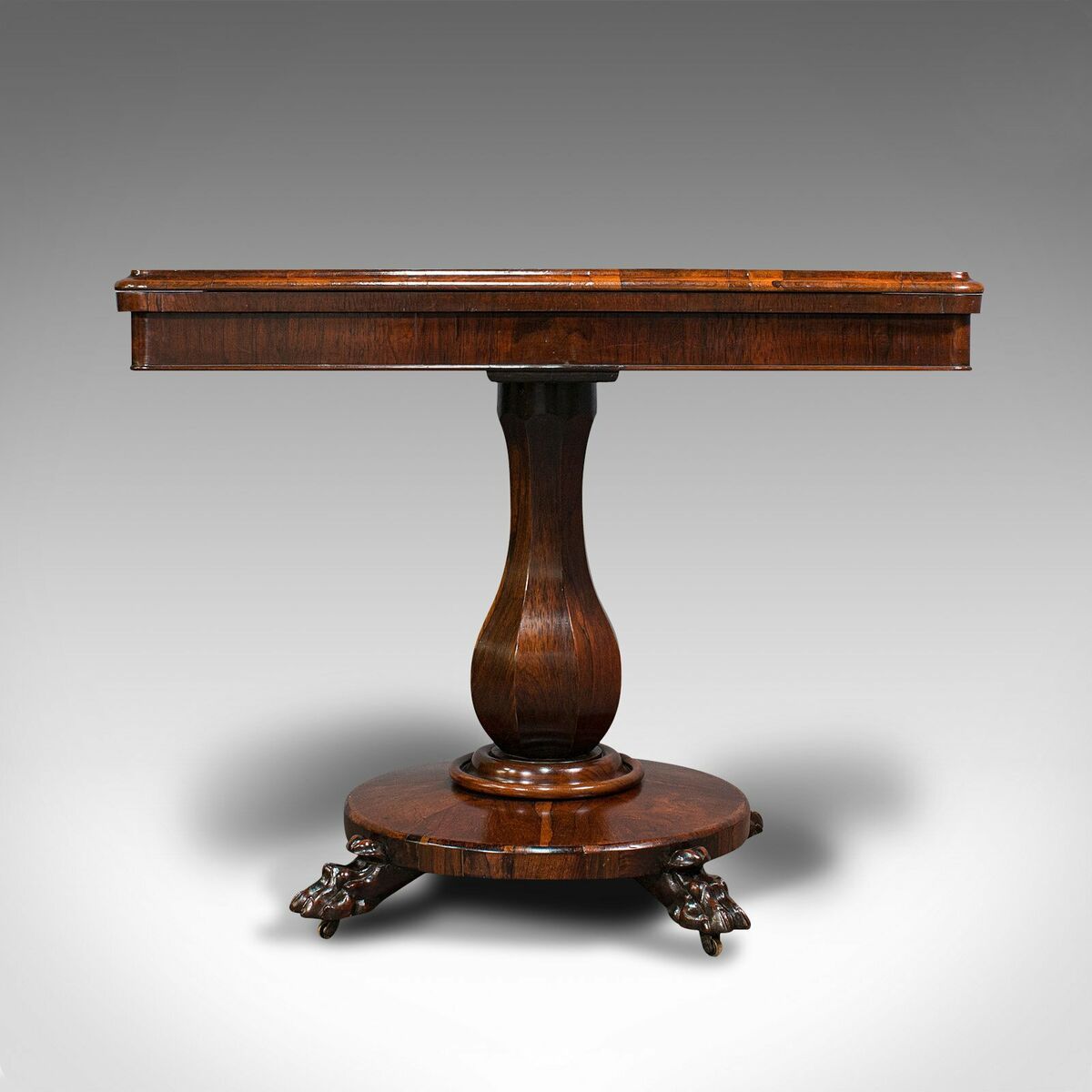This photograph showcases an antique-style poker table set against a gray, slightly illuminated background with visible shadows. The table is crafted from wood with a red mahogany stain, giving it a rich, reddish-brown hue. The tabletop is rectangular and relatively flat, about a couple of inches thick, and features a subtle lip extending around its edge.

The table is supported by an elaborate, antique base. The base starts with a round, ornately carved wooden disk, from which four intricately designed feet protrude. These feet, visible in the front, project outward and are detailed with small nubs at their ends for additional support. Rising from the center of this disk is a column that mirrors the appearance of a vase—it starts wide at the bottom, narrows as it rises, and then flares out slightly again towards the top, creating a graceful, elegant profile. The entire piece has a polished, shiny finish, highlighting the craftsmanship and intricate details.